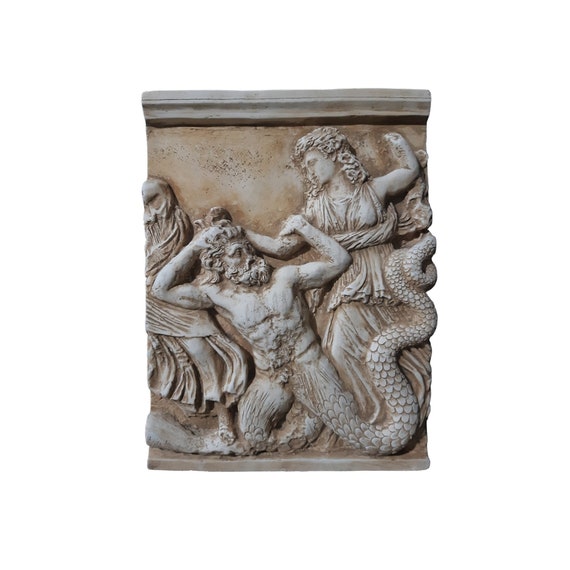This image showcases a detailed stone carving, likely a fragment from an ancient column, possibly of Greek or Roman origin. The sculpture depicts a man with long hair and a long beard, who intriguingly has the tail of a serpent or a mermaid instead of legs. His arms are raised above his head in a dramatic pose. Next to him, a woman with shoulder-length hair, dressed in a flowing garment, stands with her arm raised, seemingly about to strike him while her other hand grasps his head. Her aggressive stance suggests a dynamic interaction between them. The stone appears aged, showing slight yellowing, and hints at being part of a larger scene with additional characters that are not fully visible in this image.